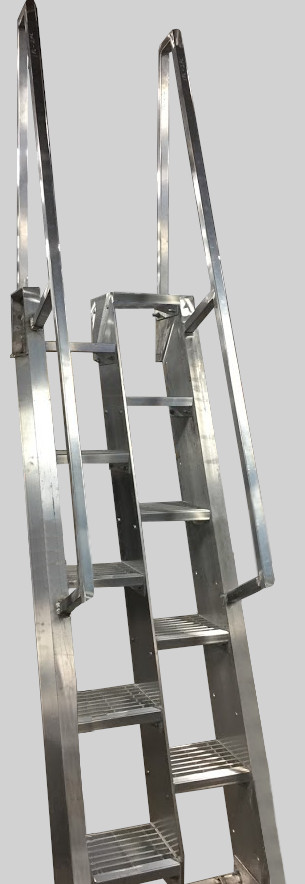The image depicts a narrow, high, industrial ladder made entirely out of silver metal, likely aluminum. The ladder features staggered steps, each step presenting a different height for the left and right foot, separated by a central metal barrier. This gives the impression that as you ascend, your feet alternately step higher and lower. The ladder is also equipped with two handlebars that begin a little below the center of the image and extend to the top, resembling the handrails found on pool stairs. The background is a light gray wall, enhancing the reflective quality of the metal. Overall, the ladder includes around ten to eleven very thin steps and seems designed for a specialized industrial or mechanical use.